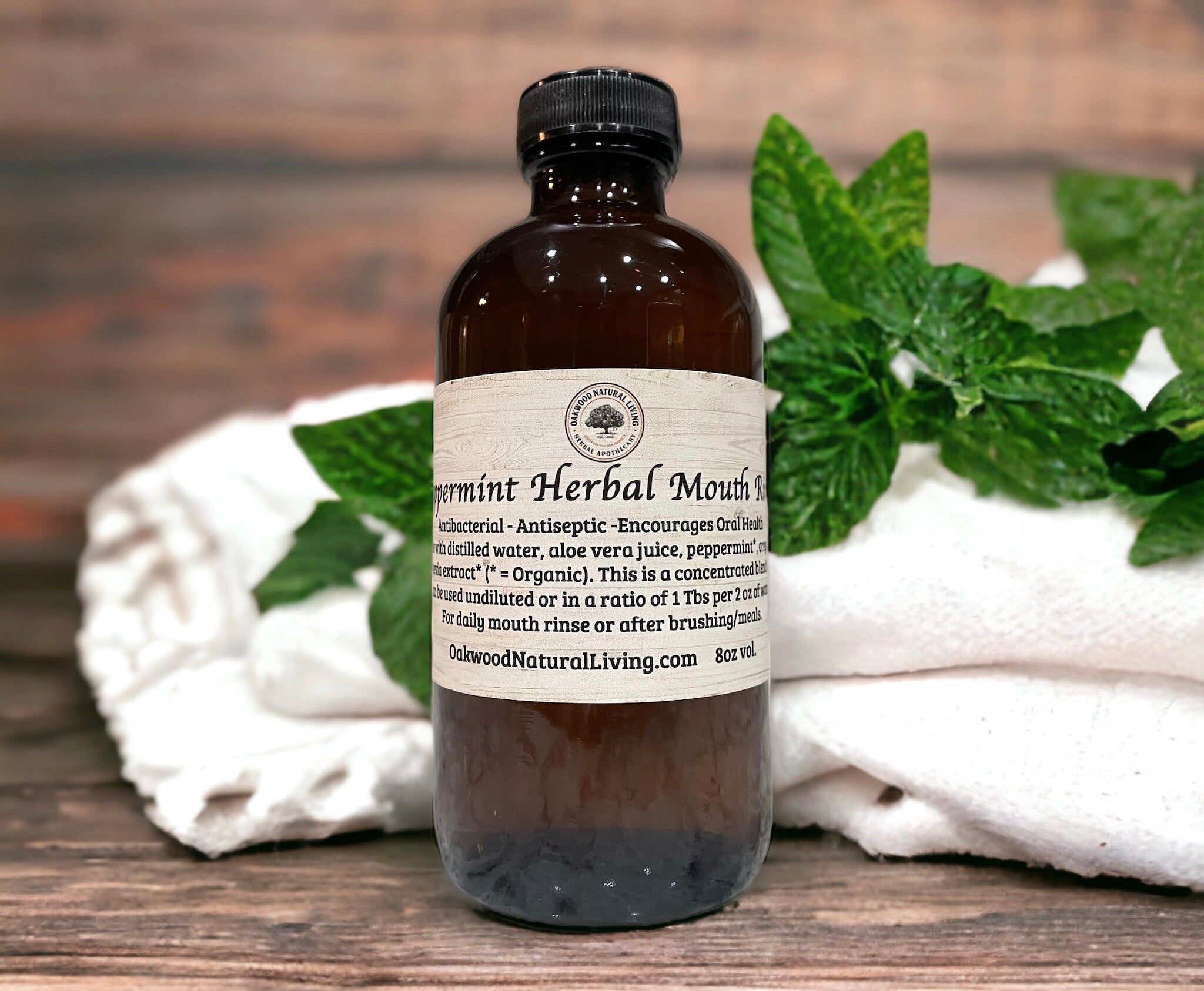The image features a dark brown glass bottle with a shiny surface reflecting white lights at the top. The bottle is topped with a black plastic cap and adorned with a white wood-grain label. The label prominently displays a circular logo reading "Oakwood Natural Living." While some of the text is partially obscured, it clearly identifies the product as a "Peppermint Herbal Mouth Rinse." Additional details on the label mention it is antibacterial, antiseptic, and promotes oral health, with ingredients including distilled water, aloe vera juice, and peppermint.

The product is described as a concentrated solution meant to be diluted at a ratio of one tablespoon per two ounces of water for daily mouth rinse use or after brushing meals. The bottom of the label includes the website "oakwoodnaturalliving.com" and specifies an 8-ounce volume. 

In the background, there are neatly folded white towels with fresh mint leaves spread on top, all set against an out-of-focus wooden backdrop, which matches the wooden surface on which the bottle is placed. This context adds a natural, clean aesthetic to the composition, highlighting the organic and herbal nature of the product.